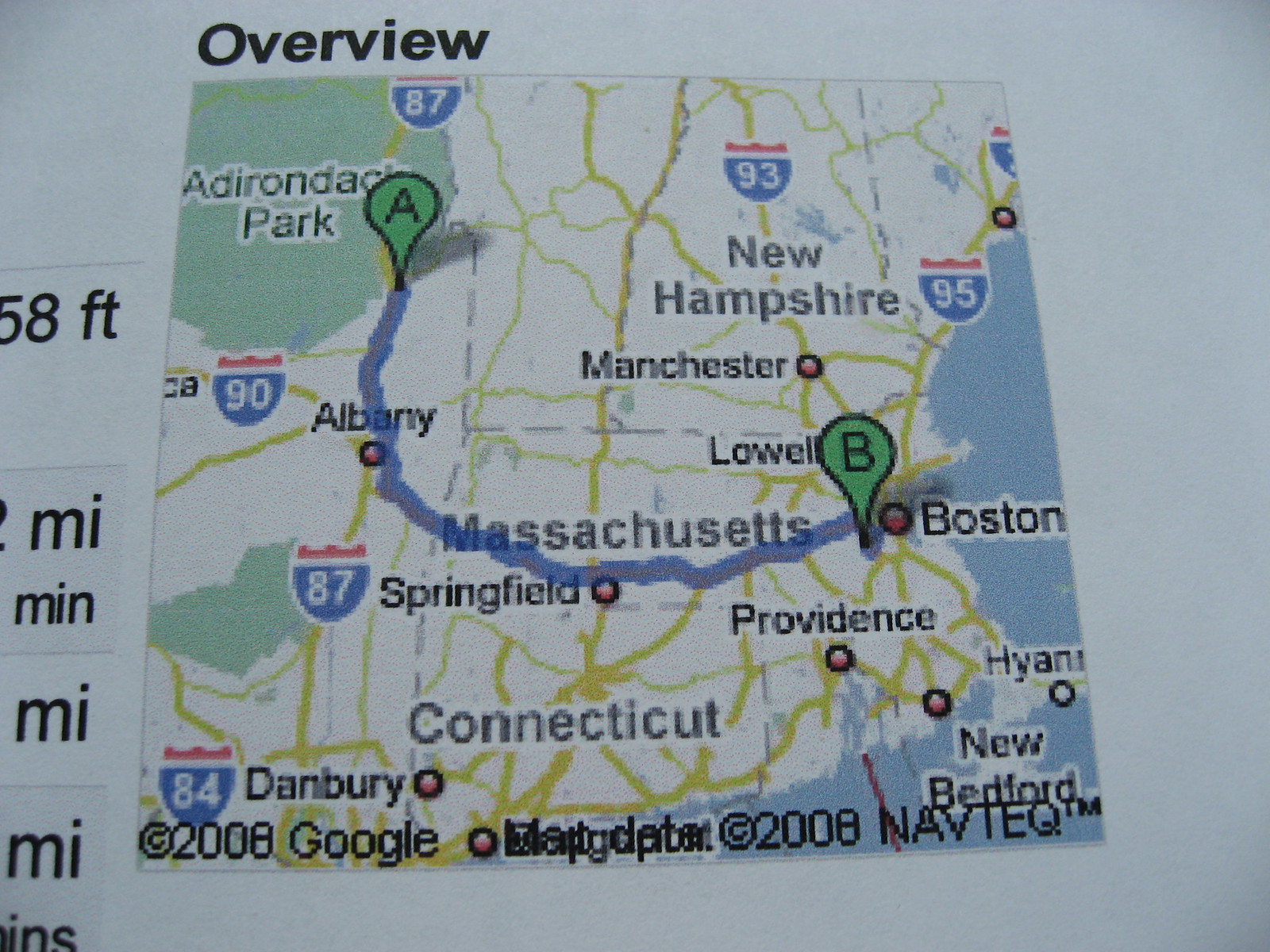The image is a photo of a computer screen displaying a map primarily of the northeastern United States, focusing on an area that includes Massachusetts, Connecticut, New Hampshire, and parts of New York. The map features a light blue or gray background with white to represent the states and blue for water bodies. At the top left corner, there's a black label reading "Overview." The map highlights a specific route from the Adirondack Park region heading towards Boston, marked with a blue line. Surrounding the route, you can see various interstates like I-90, I-87, I-84, I-93, and I-95, displayed in blue and red. Prominent locations such as Albany, Springfield, Lowell, Manchester, Providence, Danbury, New Bedford, and Boston are marked. On the left side of the screen, there's a section that provides turn-by-turn navigation details and mileage information. The map, dated "2008 Google," is a compact, website-based navigation aid showing a particular journey and its key waypoints across major interstates and cities within the region.